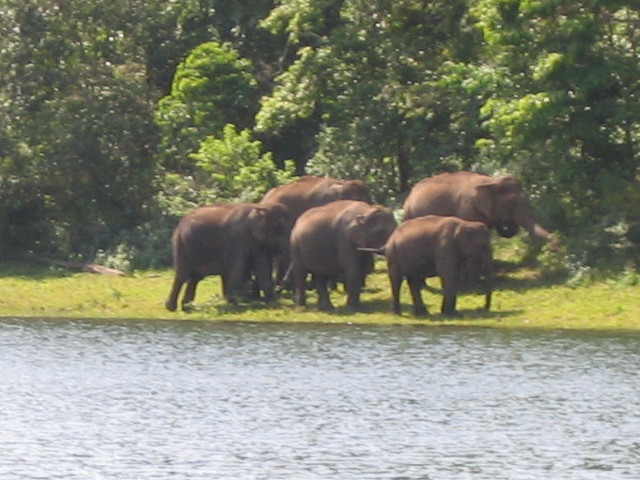In this photograph, a group of five chocolate brown elephants are walking along a grassy area next to a waterway, which appears gray with darker shades near the shoreline. The elephants' elongated trunks are all down, except for one on the right side that is exploring a nearby plant. The group is arranged with three elephants closely together in the front, followed by two slightly larger elephants behind them, possibly indicating different ages within the group. They are all moving towards the right side of the image, casting shadows due to the sunlight coming from the left. The background features a dense line of tall, deciduous trees with leaves varying from dark to light green. The scene captures an outdoor, natural setting with a slight blur, suggesting it might have been taken with an older or less advanced camera, giving the image a softer, less defined quality. The waterway, possibly a lake or pond, also shows subtle ripples under the sunny sky.